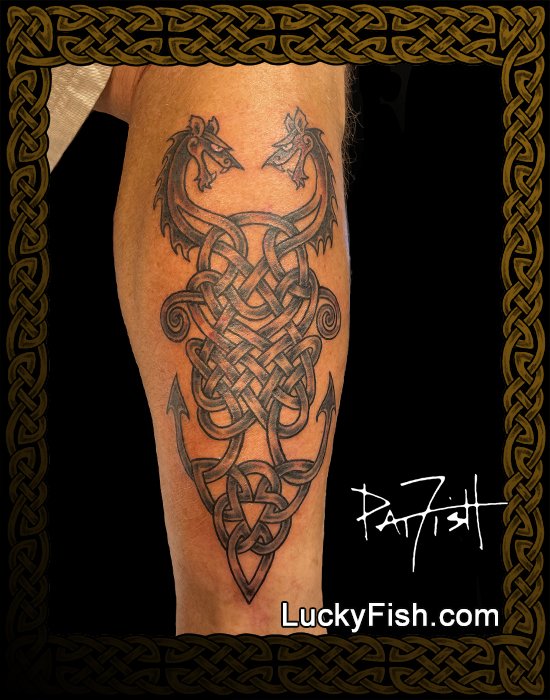The image is a vertical rectangle with a dark black background. Framing the image is a rich, dark brown Celtic weaving pattern that borders the entire picture. Centered in this design is a detailed, intricately tattooed limb, depicted either as a leg running from the ankle to below the knee, or an arm from the middle to the wrist, showing a light-skinned person wearing a beige shirt. The tattoo is an elaborate black ink design featuring two dragons entwined in a complex, woven pattern. At the top, the dragons face each other with open mouths, their bodies interlacing into a sinuous, ribbon-like motif. Lower down, their tails loop into a U-shape, converging with a simplistic triangular woven shape right above the base. The tattoo is predominantly black with some shading, and a hint of red coloring on one of the dragons. White text at the bottom right corner of the image reads "Luckyfish.com," accompanied by what appears to be the signature "Pat Fish" or "P7TISH."